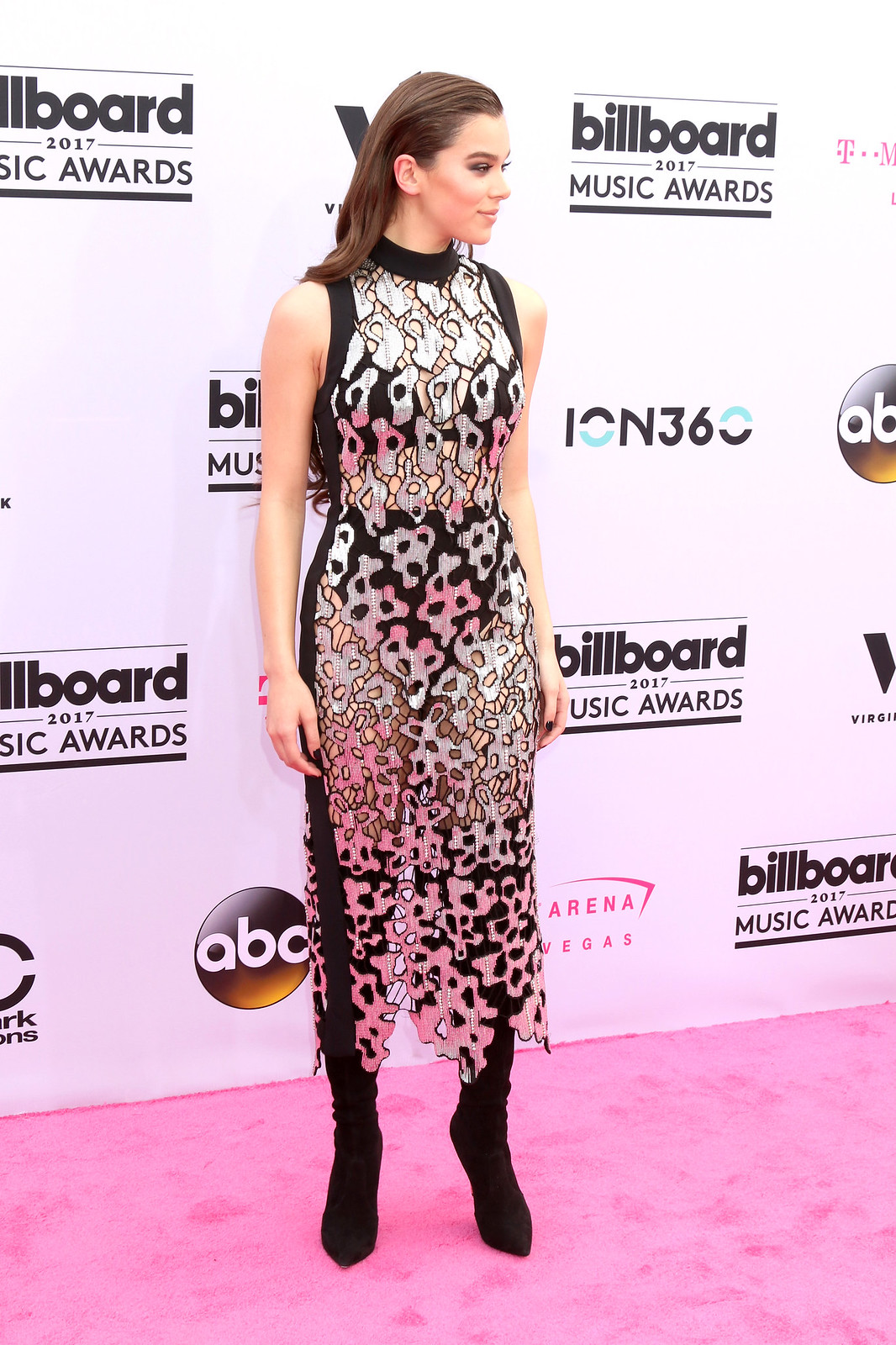In this image, a woman with shoulder-length brown hair is posing on a pink carpet at what appears to be the Billboard 2017 Music Awards. She's dressed in an elegant, sleeveless gown featuring a sheer pattern of white, gold, and black that extends down to her ankles. The dress has a black collar around her neck, and underneath it, she wears a black brassiere and black panties which are visible through the dress. She completes her outfit with knee-high black boots. Her arms are relaxed at her sides, and she is gazing to her left, likely towards the paparazzi. The background is a white poster with repeating black text that says "Billboard 2017 Music Awards," along with various logos including ABC Television Network and ION360.